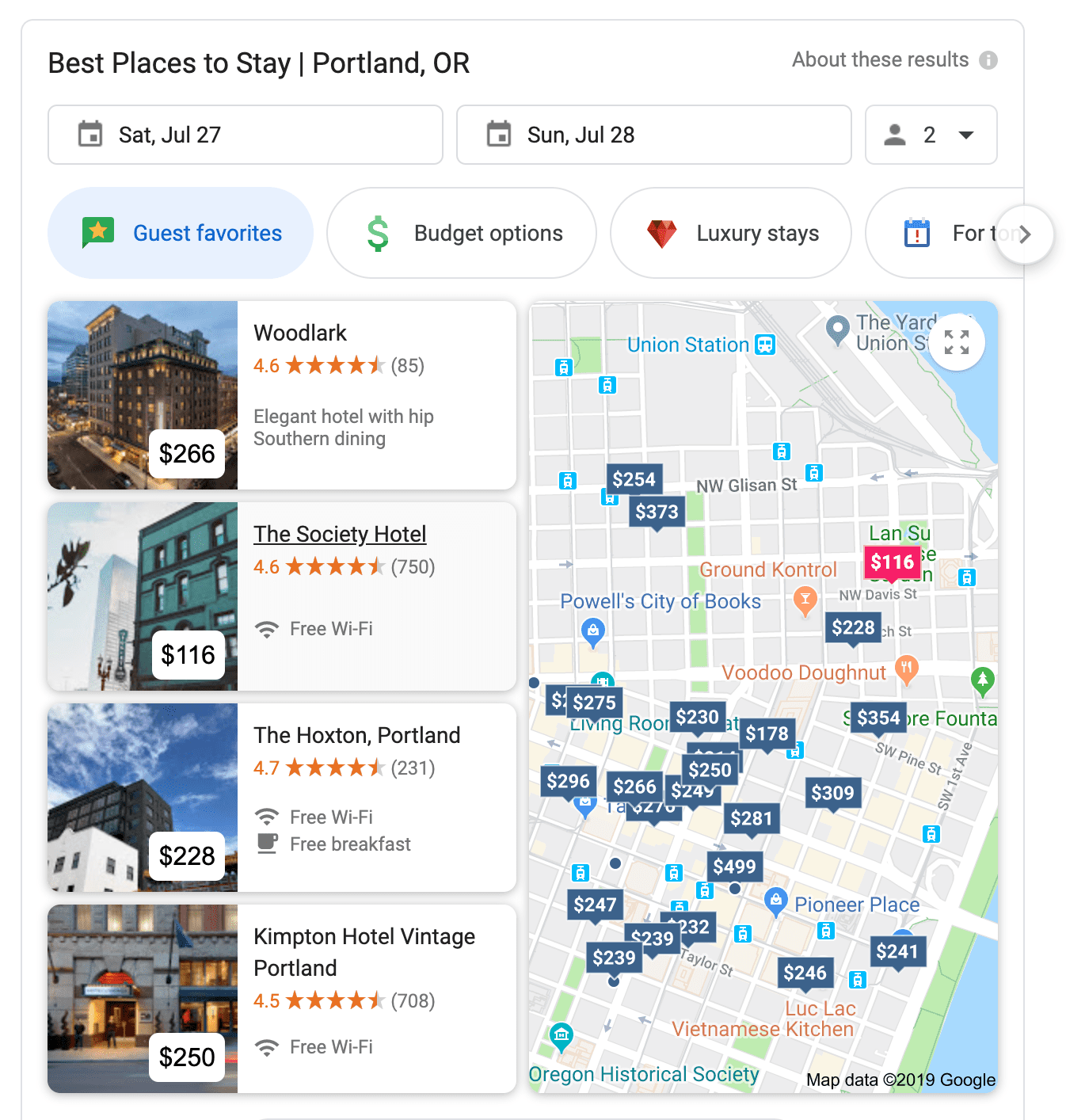This image showcases a search results page for hotels in Portland, Oregon. At the top left, the title "Best Place to Stay: Portland, Oregon" is prominently displayed. Below this, various criteria have been selected: a check-in date of Saturday, July 27, and a check-out date of Sunday, July 28. An icon of a person indicates that the search is for two guests. The "Guest Favorites" tab is highlighted, suggesting these are popular choices among travelers.

Under the tab, several hotel options are displayed with corresponding images. The first listing features an exterior shot of a large, multi-story hotel taken later in the day. This hotel is priced at $266.00 per night and is identified as "Woodlark," rated 4.60. The description highlights it as an "Elegant hotel with hip southern dining."

The second listing shows a more modern-looking hotel priced at $116.00 per night. It is named "The Society Hotel," also rated 4.60, and offers "Free Wi-Fi."

The third hotel is another modern establishment, priced at $228.00 per night. It is "The Hoxton, Portland," and it includes amenities such as "Free Wi-Fi" and "Free breakfast."

The final listing presents a close-up image of the front door and entrance area of a hotel. This hotel, "Kimpton Hotel Vintage Portland," is priced at $250.00 per night.

To the right side of the page, there is a map displaying portions of Portland with some streets labeled. Various hotels are marked on the map with blue boxes indicating their prices, helping users visualize their locations within the city.